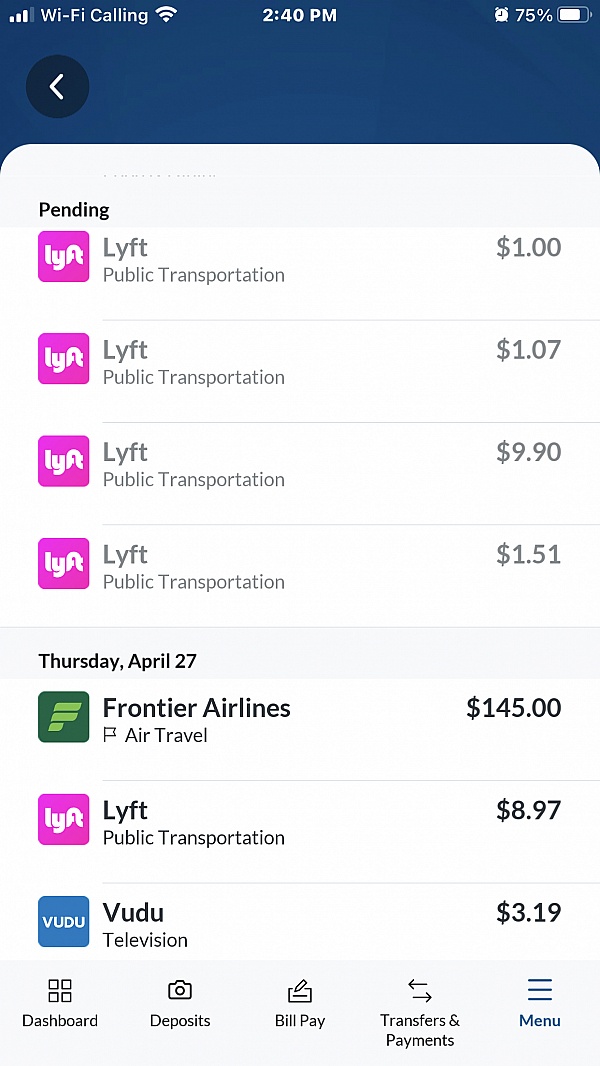This image showcases a smartphone screen featuring various transaction details on a financial application. 

- **Top Bar Details**: At the top left corner, there's a cellular signal icon followed by the Wi-Fi calling text and a Wi-Fi icon. The time displayed is 2:40 PM. Towards the top right, there’s an alarm clock icon, a battery icon indicating 75%, and a battery status image. 

- **Transaction Summary**: 
  - The first transaction marked as "Pending" features the Lyft logo and indicates a Lyft Public Transportation charge of $1.
  - The second transaction also features the Lyft logo, indicating a Lyft Public Transportation charge of $1.70.
  - The subsequent transactions repeat the same format:
    - Lyft Public Transportation: $9.90
    - Lyft Public Transportation: $1.51

- **Date and Additional Transactions**: 
  - Below these transactions, the date "Thursday, April 27th" is displayed. Adjacent to this date, there is the Frontier Airlines logo which denotes an air travel expense of $145.
  - Further transactions include:
    - Lyft Public Transportation: $8.97
    - Voodoo Television: $3.19 

- **Bottom Navigation Bar**: The bottom section of the screen features five navigation icons arranged from left to right, labeled as "Dashboard", "Deposits", "Bill Pay", "Transfers and Payments", and "Menu".

The screen's background color is primarily white, with no images or photos besides the mentioned brand logos.